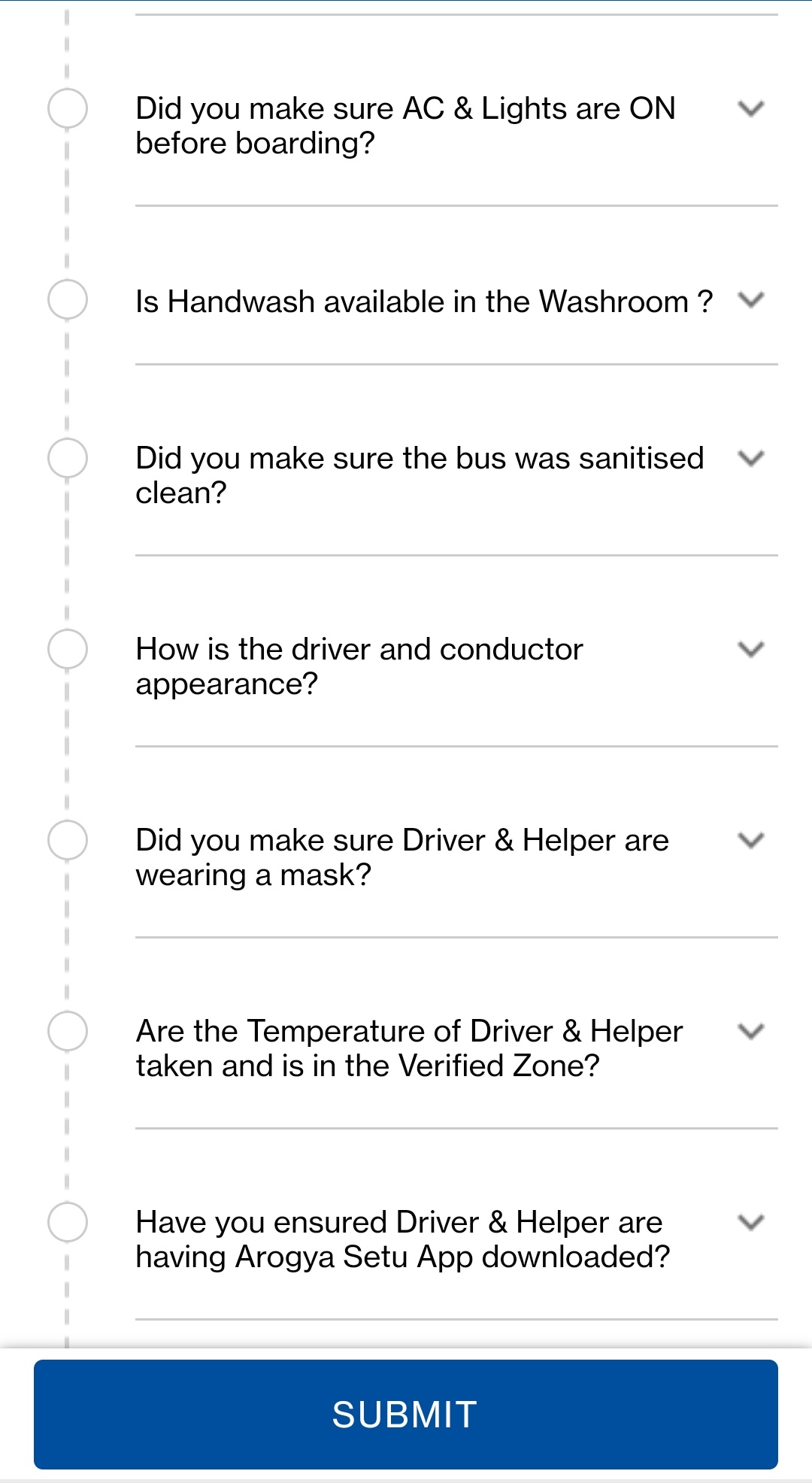**Detailed Caption:**

The image is a screenshot from an unidentified webpage displaying a detailed list of to-do items, formatted as a bullet-point list. The content appears to be a checklist for ensuring safety and hygiene protocols are met before a journey. The list begins with the following items:

1. Did you make sure AC and lights are on before boarding?
2. Is hand wash available in the washroom?
3. Did you make sure the bus was sanitized clean?
4. How is the driver and conductor's appearance?
5. Did you make sure the driver and helper are wearing a mask?
6. Are the temperature of the driver and helper taken and is it in the verified zone?
7. Have you ensured the driver and helper have downloaded the Aarogya Setu app?

At the bottom of the page, there is a dark blue rectangular button. In the center of this rectangle, the word "SUBMIT" is written in all capital letters, in white color. The image is purely textual, containing no photographs, illustrations, people, animals, birds, fish, plants, flowers, trees, buildings, signs, billboards, or automobiles. The focus is strictly on the text and the checklist details.